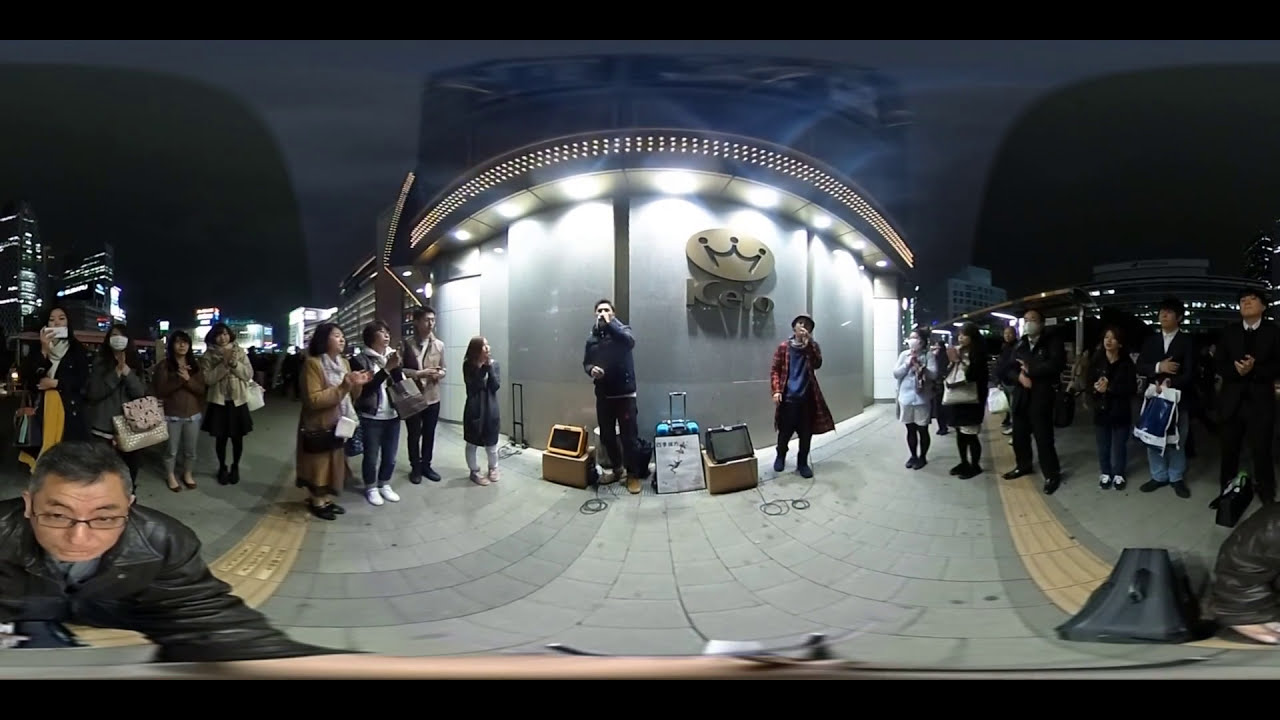The panoramic 360-degree nighttime image showcases a lively courtyard scene, where an Asian man with short, graying hair at the temples, clad in glasses and a black leather coat, can be seen prominently in the lower left foreground. His outstretched arm extends into the lower right corner of the image, indicating he might be the one taking the panoramic shot. The courtyard, paved with large gray bricks and accented by a strip of smaller yellow bricks, forms a continuous pathway extending in both directions.

At the center of the courtyard stands a gray curved building adorned with a lit marquee. The structure features a logo with a crown above the gold letters "K E I O". The building's lights, along with additional bright lights from a roofline above the performers in the middle, illuminate the entire area, giving it an almost indoor ambiance despite the clear nighttime setting depicted by the mostly black sky with dark blue clouds.

The scene buzzes with activity. A crowd of people, clad in long pants, jackets, scarves, and coats, hinting at cold weather, is gathered around two performers holding microphones. The performers are flanked by speakers, cables, and a radio, immersed in their act. Attendees are scattered throughout the courtyard, some talking on phones, carrying various kinds of luggage, and standing along the pathway.

In the background, towering buildings with their lights on add depth to the scene. The detailed lighting, the central performance, and the documented details of the environment paint a comprehensive picture of a bustling, illuminated urban night scene.